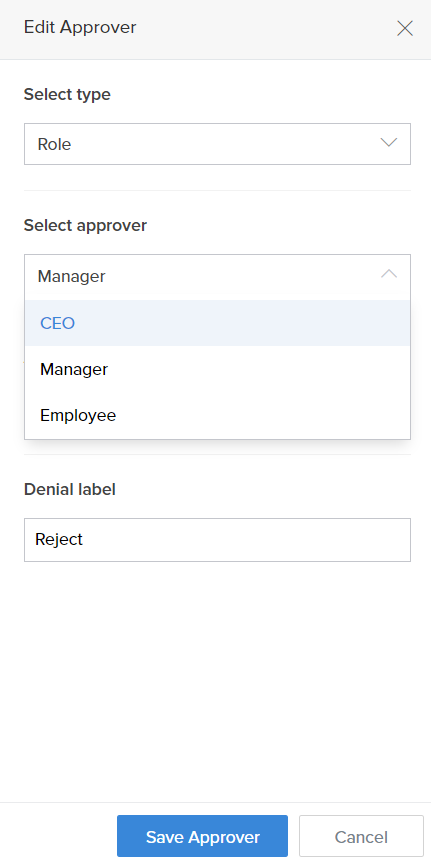The image displays a user interface featuring various pull-down menus and editable fields. At the top, there is an edit field within a grey panel labeled "Edit Approver," with an 'X' icon to the right for removal. Below this, there is a heading titled "Select Type," accompanied by a pull-down menu currently set to "Role," though its additional options are not visible as it hasn't been expanded.

Further down, another heading labeled "Select Approver" is present, featuring a pull-down menu with options including "Manager," "CEO," "Manager," and "Employee." The "CEO" option is highlighted in blue, indicating it is the selected choice.

Below, a field under the heading "Denial Label" contains the text "Reject." Beneath this series of elements are two buttons: a blue button with white text labeled "Save Approver" positioned on the left, and a white button with grey text labeled "Cancel" located to the right.